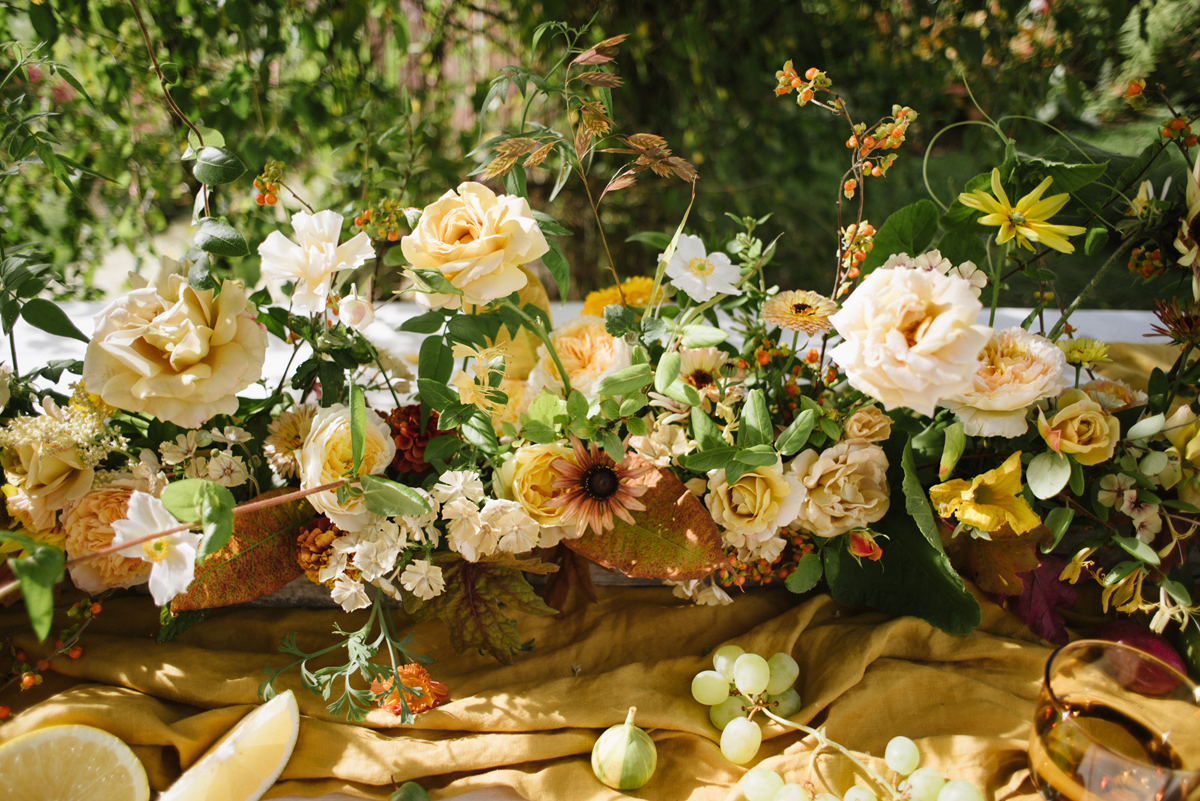This vibrant real-life photograph showcases a beautifully arranged row of diverse flowers in vivid detail. The focal point features around four or five roses in various stages of bloom, from fully open blossoms to tightly closed buds, complemented by a variety of other flowers including sunflowers, lilies, and several unidentified species. These flowers, with their lush green stems and leaves, create a dense, colorful tapestry that stretches across the image.

In front of this captivating floral display, a somewhat disheveled, yellow vintage cloth is draped haphazardly. Atop the cloth, an assortment of fruits is artfully placed, including a citric slice—potentially a lemon or an orange—a fig, a small bunch of about six grapes, and a scattering of additional grapes. A glass containing an unidentified liquid sits at the bottom right corner of the cloth, adding a touch of domesticity and balance to the scene.

Above and behind the row of flowers, the background transitions into a blur, hinting at a lush garden setting teeming with vines and greenery. The bokeh effect artfully keeps the focus on the main floral and fruit arrangement, enhancing the depth and richness of the composition while inviting viewers to immerse themselves in the serene, natural beauty of the scene.